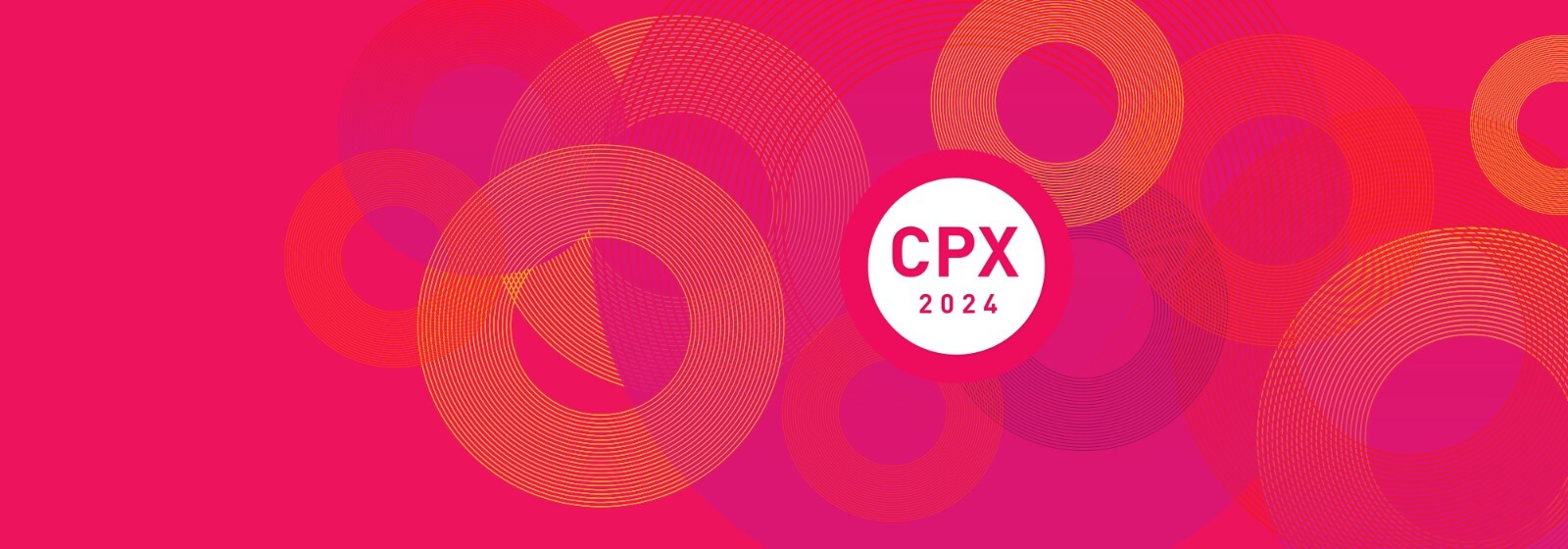The image is a vibrant, computer-generated banner featuring a small rectangle that is elongated horizontally. The main background color is dark pink, with various circles of different sizes and pastel shades, including red, purple, orange, and pale yellow, intersecting and overlapping each other across the canvas. Towards the right of the center is a prominent white circle with dark pink edges containing text. The text is in bold dark pink, displaying "CPX 2024" in large capital letters. This central lettering suggests the image is an announcement or advertisement for an event, likely a conference or a product launch. The intricate design of intersecting circles adds a dynamic and artistic flair to the overall visual.